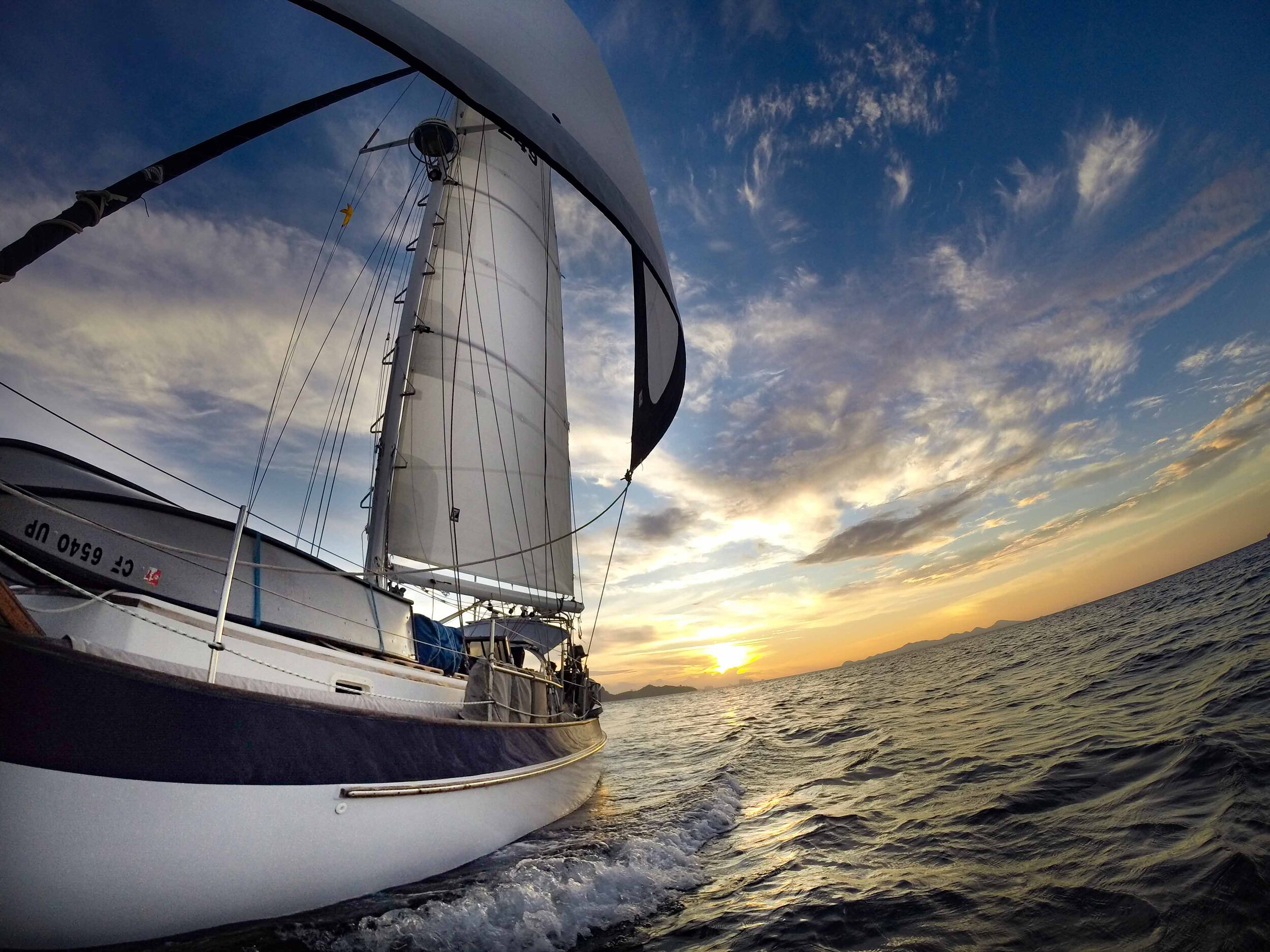A medium-sized sailboat with a white bottom and a navy-striped top cuts through the tranquil sea, creating a wake of white waves against the darkish green waters. The boat, positioned on the left-hand side of the image, features a bowed sail catching a breeze and a smaller, upside-down boat atop it marked with the letters CF650UP. The photograph, likely captured with a drone or GoPro to achieve a fisheye effect, reveals no passengers. In the background, a glowing orange sun sets, casting a band of golden light across the clear blue sky, speckled with clouds, as it approaches the horizon.